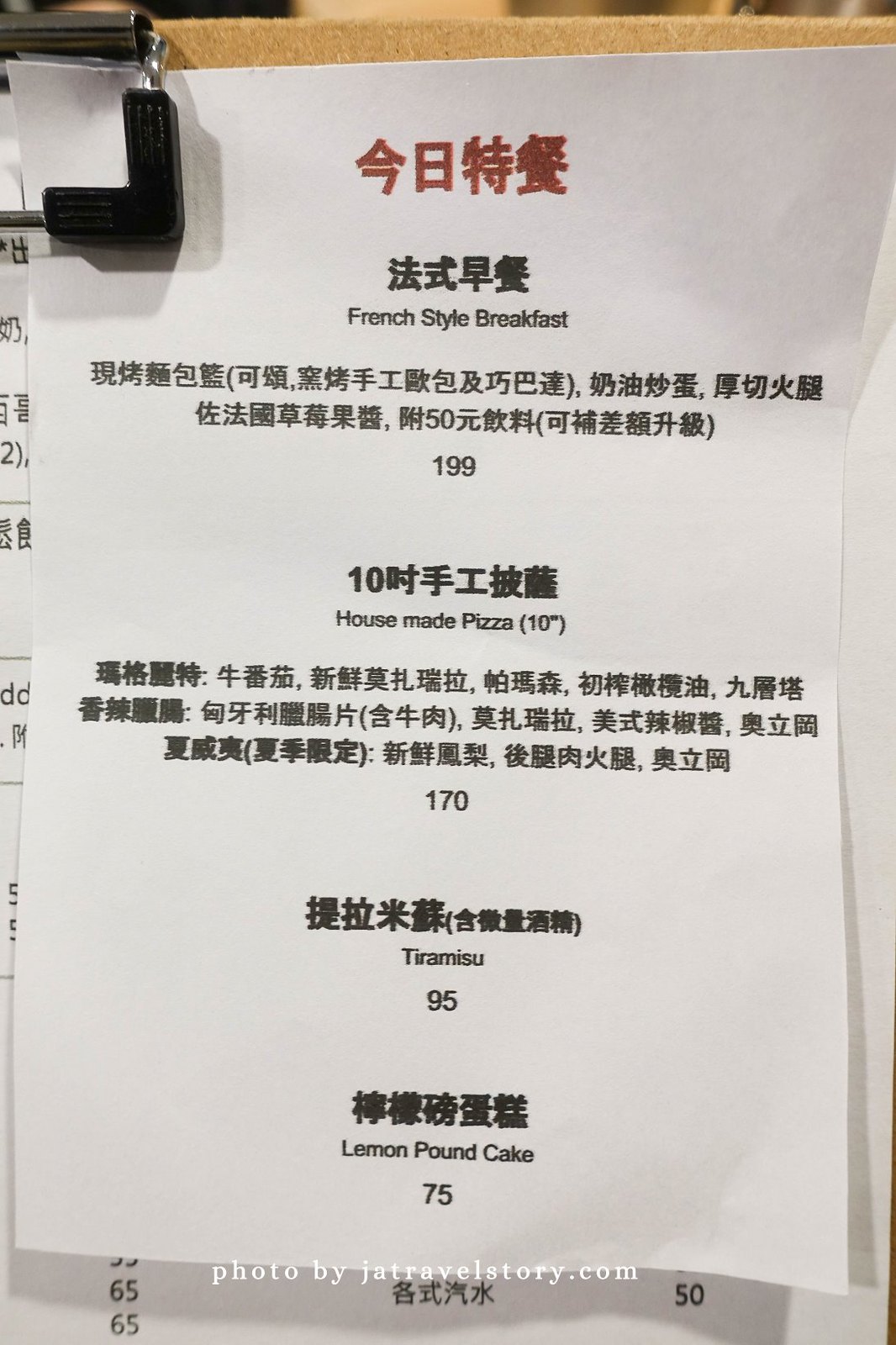The image depicts a small piece of paper, resembling a receipt or a menu, attached to a standard-sized clipboard. The paper, written in Japanese Kanji with accompanying English translations, occupies only one corner of the clipboard, highlighting its diminutive size. At the top, there's a red Kanji heading, followed by a series of menu items listed in darker ink.

Each item is presented with an English translation beneath its Kanji description. For example, the receipt lists a "French-style breakfast" priced at $1.99, a "10-inch house-made pizza" for $1.70, "tiramisu" at $0.95, and "lemon pound cake" for $0.75. Detailed descriptions accompany each item, though they are written in Kanji, making them unreadable to those unfamiliar with the language.

At the bottom of the image, a white font watermark reads "photo by JATravelsStory.com," which somewhat blends into the background, making it a less optimal choice for visibility.